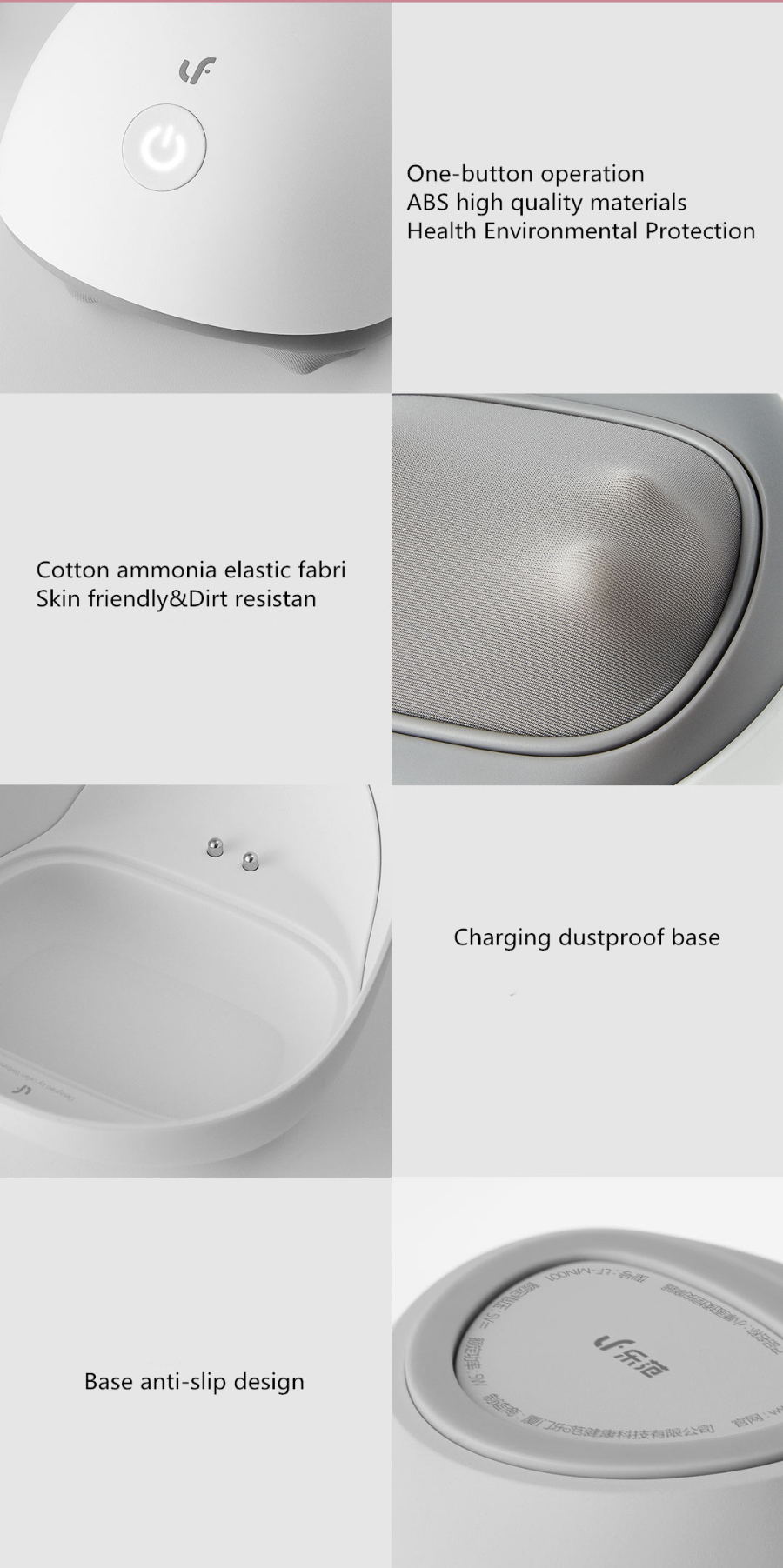The image displays a device presented through a structured layout of two columns with four boxes each. The boxes alternate between images of the device and informational text describing its features.

- The top left box features an image of a sleek white device with a prominent white power button marked with the "LF" logo.
- Adjacent to it, in the top right box, gray text highlights the device's attributes: "One button operation," "ABS high quality materials," and "Health environmental protection."
- The second row's left box contains text stating: "Cotton, ammonia, elastic fabric," and "Skin-friendly and dirt-resistant."
- The right box in this row displays an image of a textured surface resembling bumps under a cloth material.
- The third row's left box shows an image of a white area, presumably the charging station, labeled "Charging dustproof base."
- To the right, another text box describes: "Base anti-slip design."
- The bottom left box includes text about "Base anti-slip design."
- The corresponding image in the bottom right box depicts a gray base, possibly made of plastic.

The overall layout is designed to provide comprehensive information about the device, emphasizing its user-friendly operation, high-quality materials, and practical features.